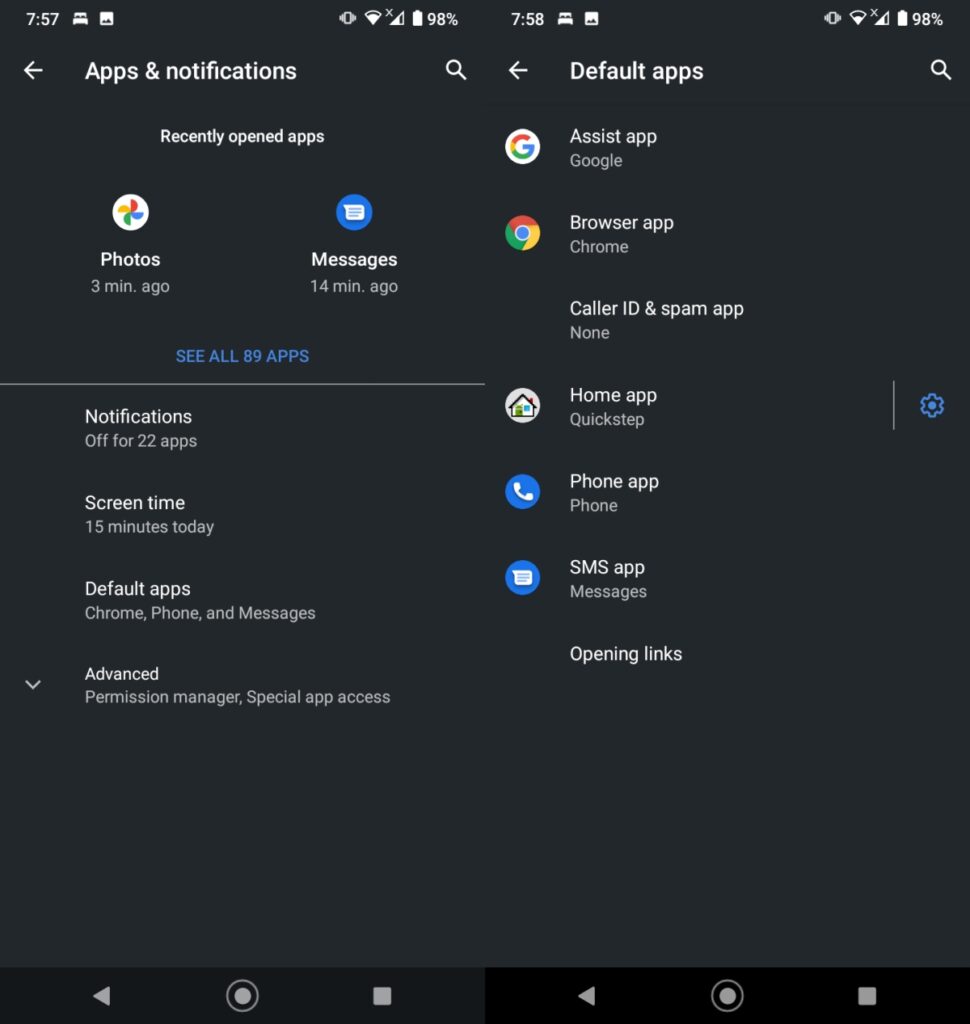The image appears to be a composite of two screenshots taken from the same iPhone, one minute apart, displaying settings related to apps and notifications.

**Left Screenshot (7:57 PM, 98% battery):**
- **Title:** "Apps & notifications"
- **Background:** Black
- **Content:** 
  - *Recently Opened Apps:* 
    - Photos (3 minutes ago)
    - Messages (14 minutes ago)
  - *Notifications:* 
    - An option to "See all 89 apps" highlighted in blue
    - Notifications turned off for 22 apps
  - *Screen Time:* 
    - 15 minutes used today
  - Sections for: 
    - Default Apps
    - Chrome
    - Phone
    - Messages
    - Advanced
    - Permission Manager
    - Special App Access (with a drop-down menu)

**Right Screenshot (7:58 PM, 98% battery):**
- **Title:** "Default apps"
- **Background:** Black
- **Content:** 
  - Listed Default Apps with their icons:
    - *Assist app:* Google
    - *Browser app:* Chrome
    - *Caller ID & spam app:* None
    - *Home app:* Quickstep
    - *Phone app:* An image of a phone
    - *SMS app:* An image of a message in blue
  - Additional icons and navigation elements such as boxes, circles, and an arrow
  
The screenshots together provide a detailed overview of the app settings and notification preferences on the iPhone.